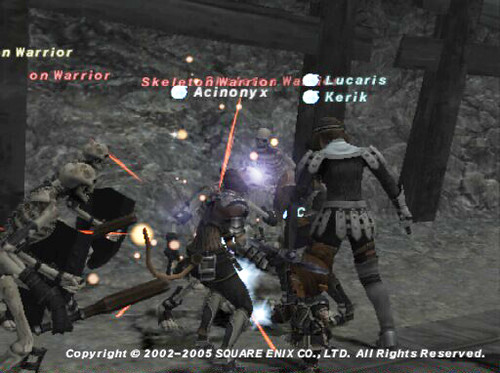This is a detailed screenshot from a medieval-themed video game, featuring a dark outdoor setting against a background of light gray rocky boulders and a wooden cross structure. The scene depicts an intense battle between characters using swords and seemingly undead skeleton warriors. The skeletons wield shields and appear to be launching an attack with red laser-like lines targeting a figure, distinct for having a tail. Accompanying this character is another, clad in historical battle gear, likely symbolizing the diversity of combatants. At the top, in yellow letters, the text reads "warrior" and "on warrior," with "skeleton warrior" mentioned below in pink. To the right, names such as "Acronox," "Lucaris," and "Couric" are labeled in white, each beside a white blotch. At the very bottom, in white lettering, there's the copyright notice: "2002-2005 Square Enix Co., Ltd. All rights reserved." This captures the essence of mid-2000s fantasy role-playing games with a combination of intricate character details and dynamic battle elements.